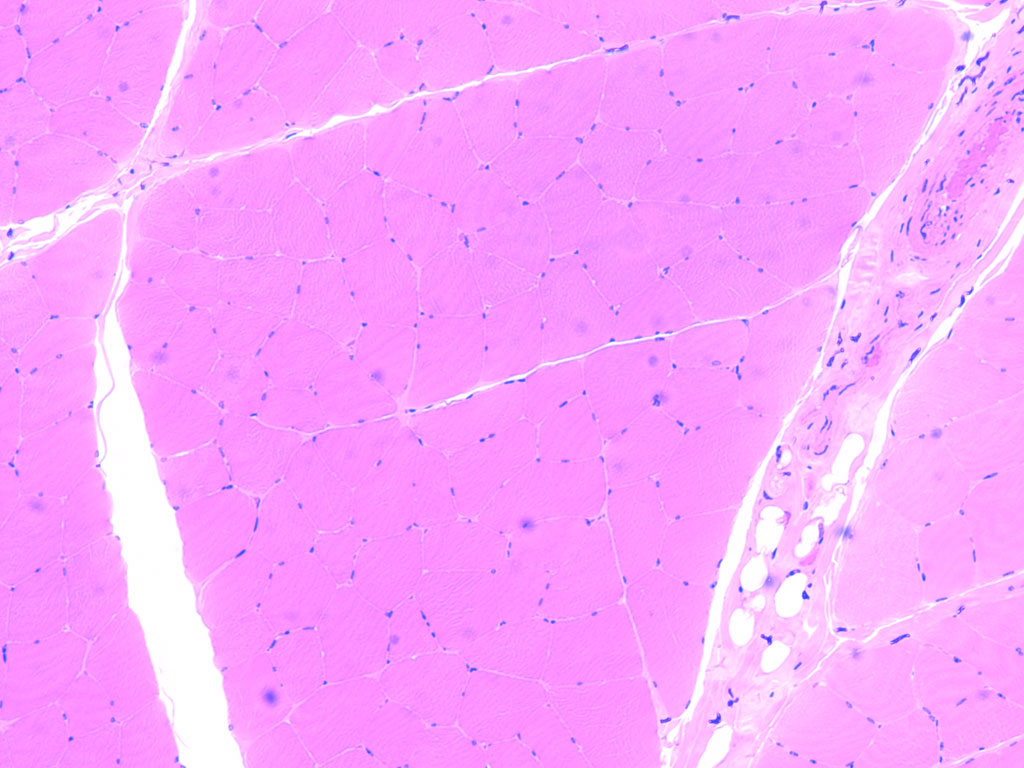The image presents a microscopic close-up of what appears to be cellular structures. The predominant colors are shades of pink and purple, giving the entire image a pastel hue. Scattered across the background are numerous darker purple dots and patterns, indicating detailed cellular components. Intersecting the pink and purple background are several white lines: one extends from the top to the bottom of the image, expanding towards the bottom; another stretches from the left side to the top right corner; and a third runs from the top right corner to the bottom. These white lines are thin and weave through various parts of the image, creating a network-like appearance. Additionally, there are two prominent white streaks on either side of the image; the one on the left is purely white, while the one on the right has a faint pink overlay. Interspersed among these lines and streaks are large, interconnected masses with triangular, squared, and rectangular shapes, contributing to the intricate and complex cellular landscape displayed in this close-up photograph.